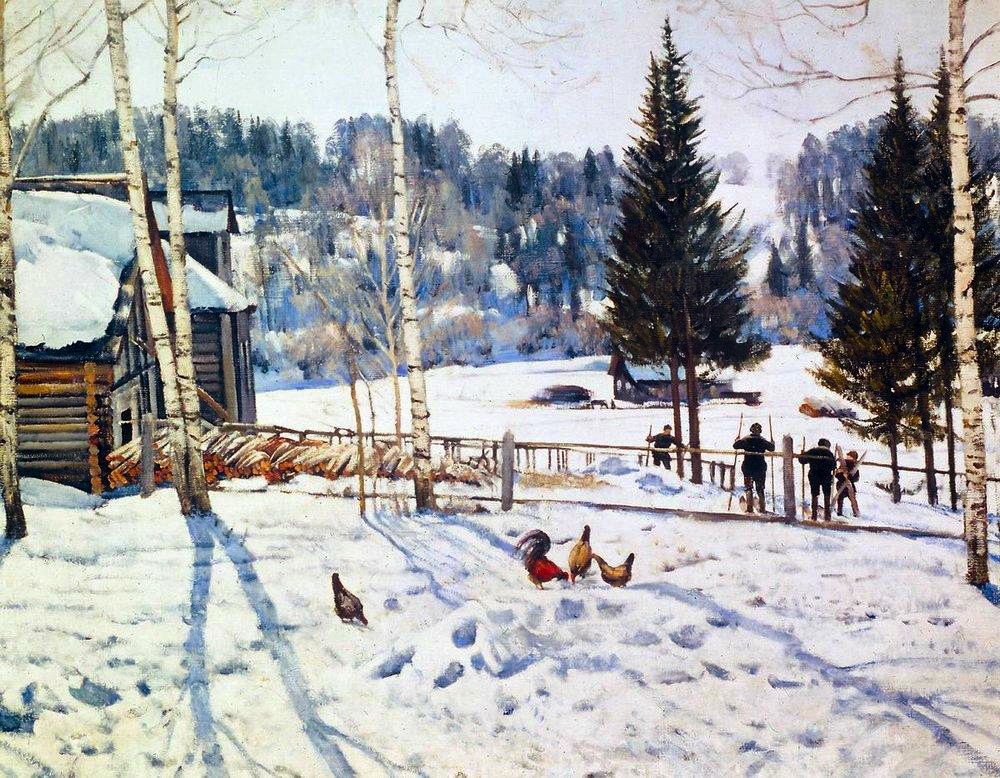The image is a square painting depicting a serene, snow-covered outdoor scene with a log cabin to the left. The cabin, intricately detailed with different shades of brown, is laden with blankets of white snow. One visible window peers out onto the wintry landscape, and a fence stretches from the cabin across the canvas, connecting the elements of the scene. In the foreground, amidst the pristine snow, footprints punctuate the landscape, leading to three chickens and a bright red rooster pecking at the ground. The chickens vary in color, with browns and lighter hues.

Standing near the fence are four people, possibly engaged in activities such as skiing or wood collecting, dressed in black jackets and pants. One of them, a child, is holding skis. Behind them, the snow-laden ground extends to the distant background, where another cabin can be seen, dwarfed by the numerous tall, narrow trees with bare branches. Evergreen trees, resembling Christmas trees, add depth and texture to the scene, particularly clustered around the people and in the upper portions of the painting.

Above, the sky is a gentle gradient of light gray and white, blending seamlessly into the frosty atmosphere. The entire composition suggests an old-fashioned, antique aesthetic, capturing a quiet winter morning or day in exhaustive detail, where every element—from the structures to the people and animals—interacts harmoniously within the cold, tranquil beauty of this rural landscape.